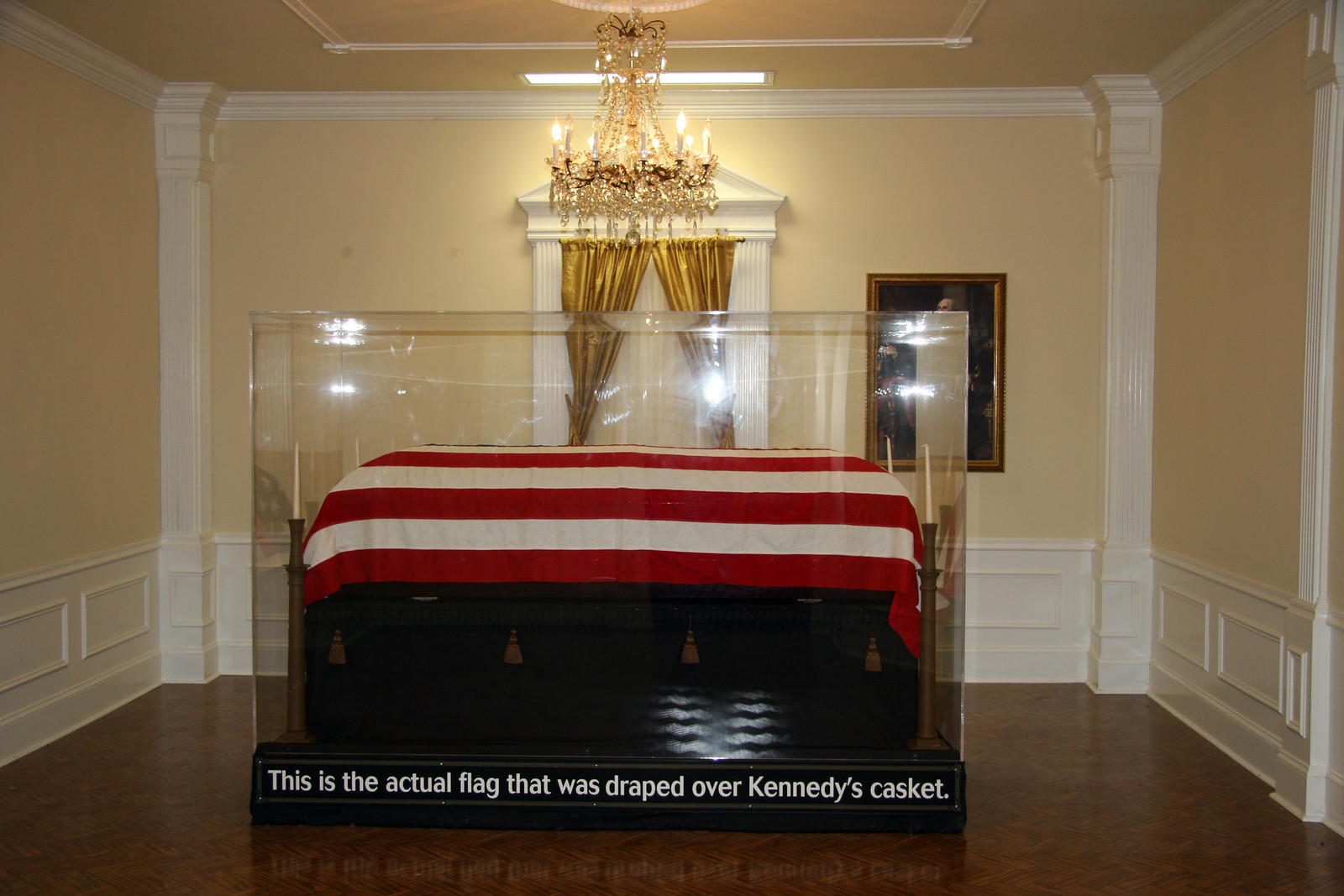The image depicts a formal room that likely belongs to a museum dedicated to President John F. Kennedy, possibly situated in Washington, D.C. or a significant historical building like the White House. The walls are painted a soft yellow hue, bordered with white crown molding and wainscoting at the bottom. Thin white columns frame the room, adding to its elegant ambiance. From the middle of the ceiling, a grand gold chandelier hangs, adorned with candle-shaped light bulbs that illuminate the space. 

The centerpiece of the room is a clear glass case placed on a polished dark wood floor. Inside the case lies a black casket draped with the American flag, historically significant as it was used to cover President Kennedy's casket after his assassination. The base of the display features a black horizontal plaque that confirms the flag's authenticity. 

At the back of the room, gold curtains are parted on either side of a white door frame, accompanied by a gold-framed picture, obscured partly by the display. In the upper right corner of the room, there's another picture, potentially of George Washington. The overall setting emanates a sense of solemn reverence and historical significance, befitting the memory of President John F. Kennedy.